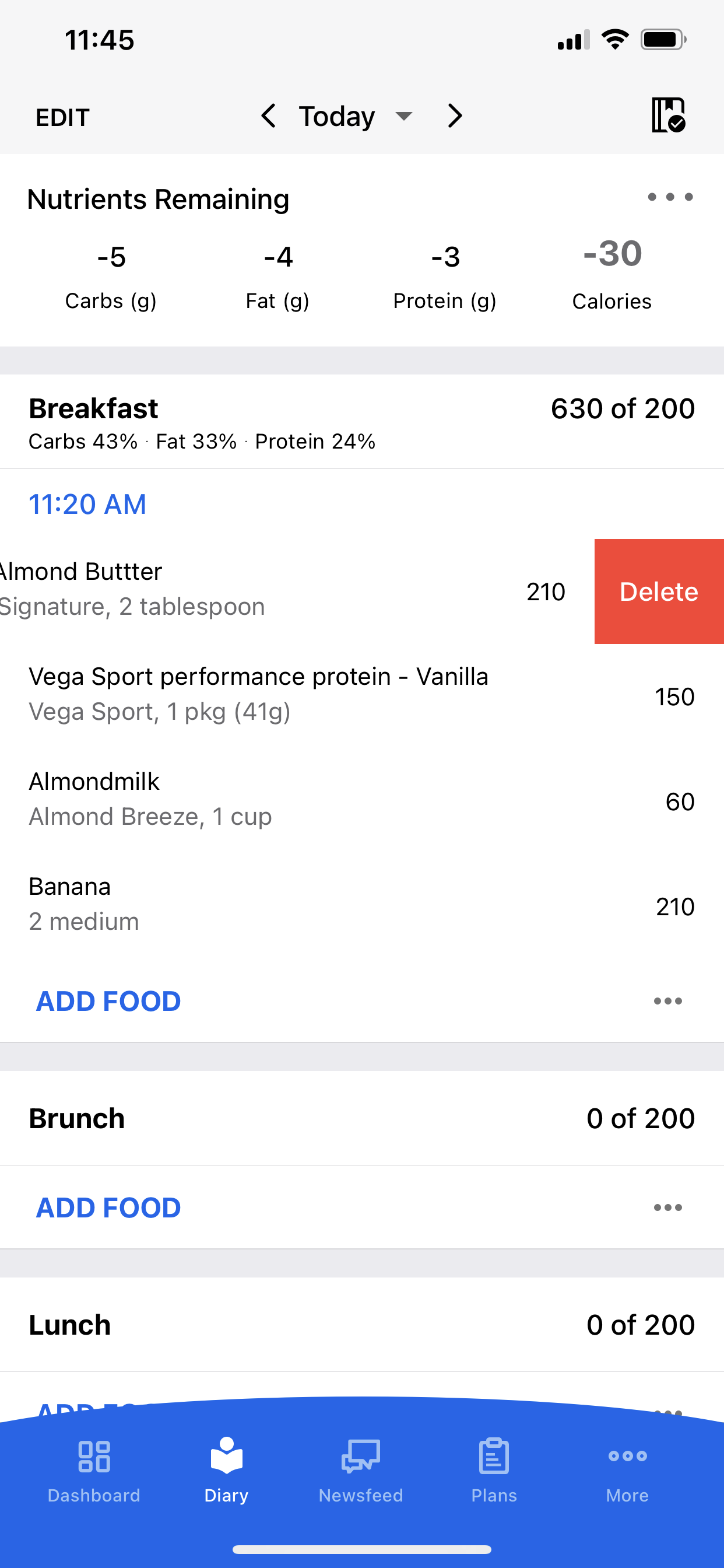The image depicts a smartphone screen displaying a nutrition tracking website. The phone's status bar indicates a nearly full battery, a strong network connection, and the time as 11:45. At the top, there is an "Edit" option. Centrally, the screen features the text "Today" accompanied by a drop-down box and navigation arrows on either side.

The section titled "Nutrients Remaining" shows the following values as negatives: carbs -5, fat -4, protein -3, and calories -30. A gray bar labeled "Breakfast" illustrates detailed consumption information, indicating a total of 630 out of 200 units (an apparent discrepancy), with macronutrient breakdowns: carbs at 43%, fat at 33%, and protein at 24%. 

The logged items for breakfast include:
- Almond Butter Signature: 2 tablespoons, 210 calories (delete option in red)
- Vega Sport Performance Protein Vanilla: 1 package, 150 calories
- Almond Milk: 1 cup, 60 calories
- Banana: 2 medium, 210 calories

There is a blue "Add Food" button beneath the breakfast details.

Following this, the "Brunch" section is empty, displaying 0 out of 200 units, with another "Add Food" button beneath it. Similarly, the "Lunch" section shows 0 out of 200 units with an option to "Add Image".

At the bottom of the screen, a navigation bar features various options: "Dashboard," "Diary," "Newsfeed," "Plans," and "More."